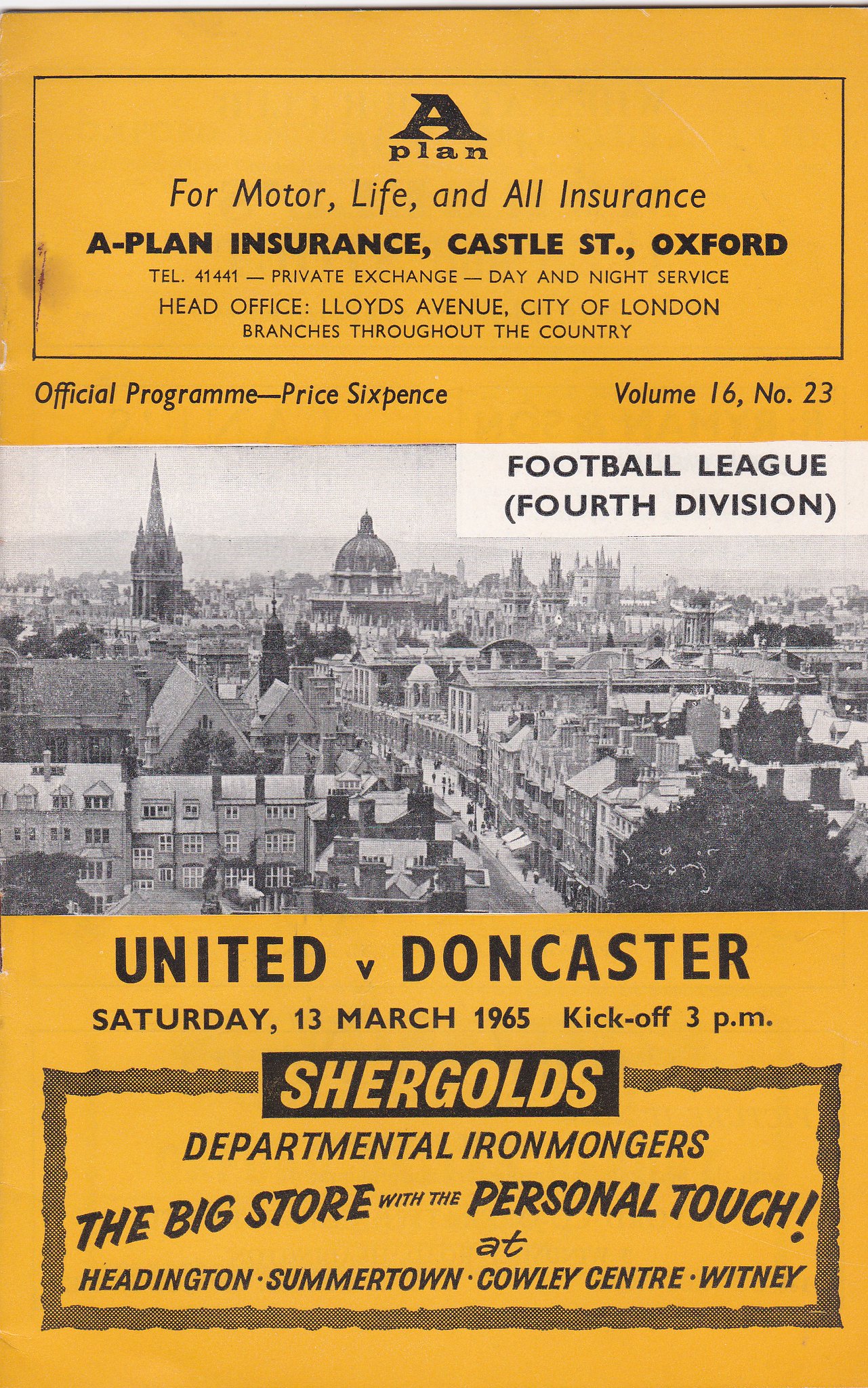This detailed image depicts a vintage pamphlet cover from 1965 printed on orange paper, primarily in black text. At the top, an advertisement for A-Plan Insurance reads, "A-Plan for Motor, Life, and All Insurance, A-Plan Insurance, Castle Street, Oxford, Telephone 41441, Private Exchange, Day and Night Service, Head Office, Lloyds Avenue, City of London, branches throughout the country." Below that, it states, "Official Program - Price Sixpence," and identifies itself as Volume 16, Number 23. 

The central portion of the cover features a black-and-white photograph of a crowded city skyline, showcasing buildings and dome-shaped landmarks, suggesting a European, likely British, setting. Overlaid on the photo in a white box, the text reads, "Football League (4th Division)." 

The bottom third of the pamphlet announces a football match, "United vs. Doncaster, Saturday, 13th March 1965, kick-off 3pm." Below this, a further advertisement for Shergold's Departmental Ironmongers states, "Sharegolds, the big store with a personal touch," listing locations in Heddington, Rivertown, Cowless Centre, and Whitney.

Overall, the pamphlet exudes a vintage print style, reminiscent of mid-20th-century design.